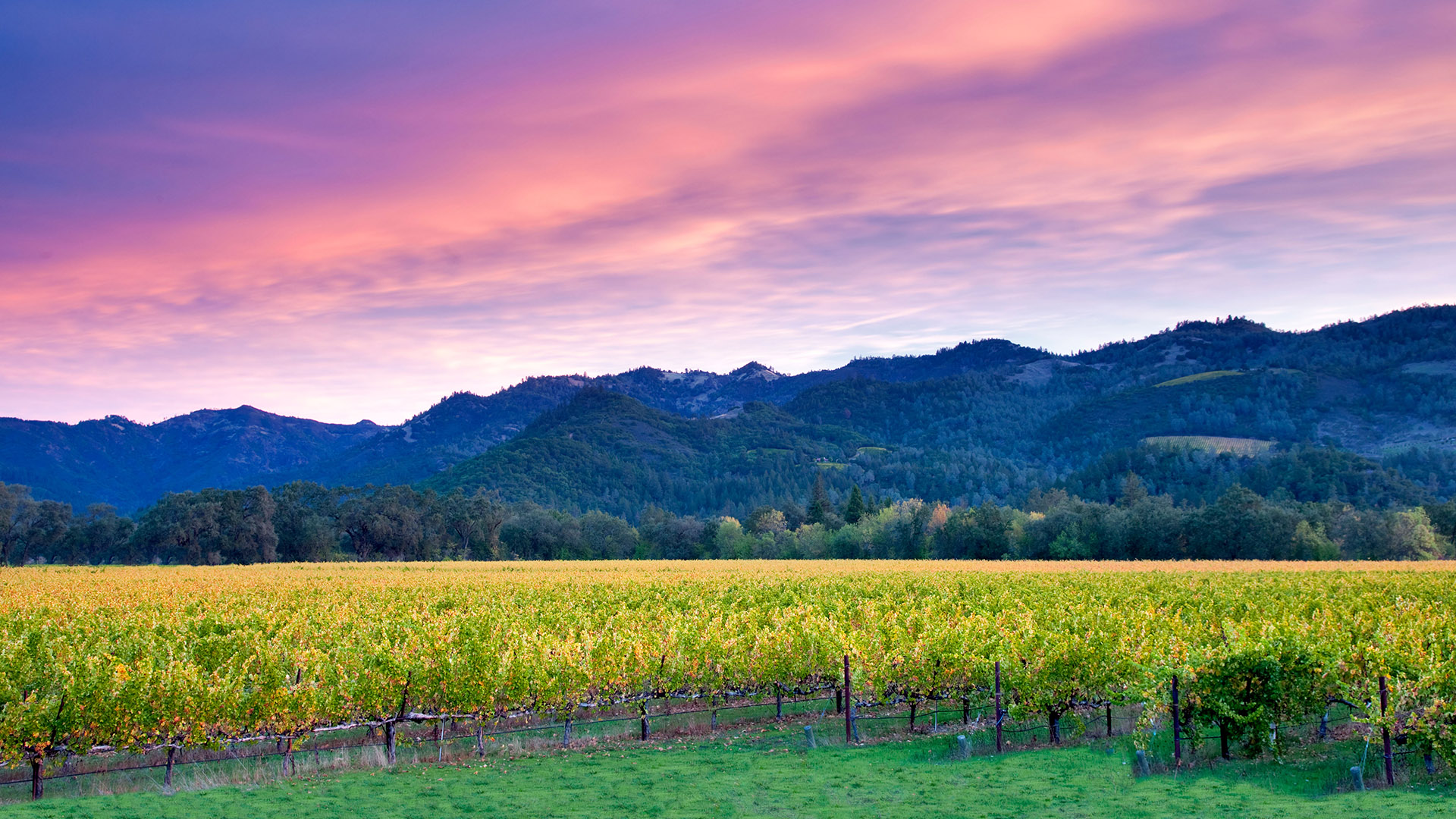The image depicts a tranquil natural landscape featuring a wide, green field, possibly filled with wheat or another uniform type of plant. The perspective appears to be from a slight elevation, roughly one story high, providing a comprehensive view over the field. Along the bottom edge of the field, there is a mix of grass and rows of yellow flowers adding vibrant detail. Beyond this field, a dense forest line extends into rolling hills which appear bluish due to atmospheric lighting. These hills rise further into the background, merging into a series of mountains that are characterized by their blue and purple hues. The mountainsides are densely forested with trees. Above all this, the sky presents a picturesque, transitioning from blue to purplish-pink tones, indicative of a setting sun, and is adorned with wispy, white clouds. The scene evokes a sense of serenity and untouched wilderness, suggesting an isolated, peaceful location far from civilization.